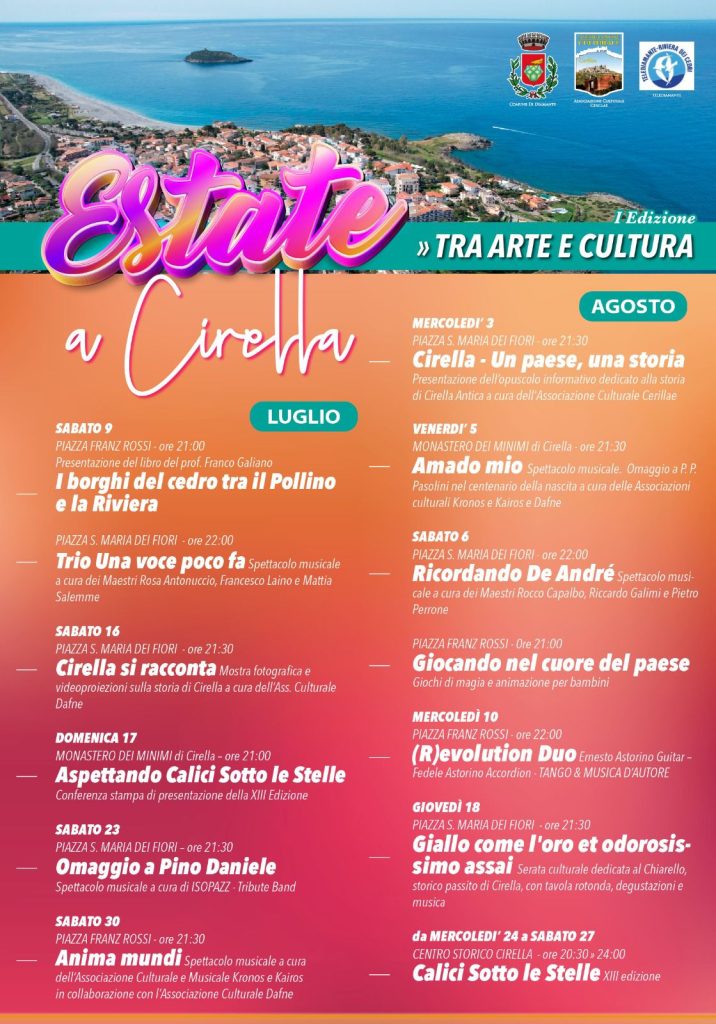The image features a large travel brochure with a stunning aerial view of a seaside community at the top, showcasing a beautiful blue ocean, sandy beaches, and a small village, likely during a sunny spring or summer day. Prominently, in bright pink and cursive lettering, the word "Estate" appears, accompanied by the phrase "Trae Arte y Cultura" in white font to its right. The brochure’s background transitions from a vivid orange at the top to a deep red towards the bottom. Scattered throughout are numerous bullet points in white font, listing various activities, schedules, attractions, dates, and locations—all written in Spanish—promoting this vibrant tourist destination.